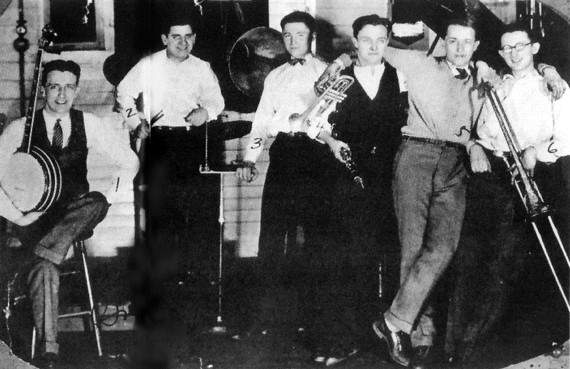This is an old black-and-white photograph that appears to have been taken in the early 1900s. It features six musicians, five standing and one sitting on a stool on what looks like a stage with a brick wall backdrop. The man on the far left is seated and holding a banjo. To his right, there is a man standing next to a drum, holding drumsticks. The remaining four musicians to the right appear to be holding brass instruments; from left to right, they include a man with a clarinet, another standing next to a tuba, a man with his arms around the men on either side of him holding a trumpet, and the man on the extreme right holding a tuba. They are dressed in white shirts, some with vests, and at least two are wearing ties. The group exudes a sense of camaraderie and joy, giving off a speakeasy vibe. There are numbers written on each of the men, with 'one' on the third from the left and 'six' on the far right.